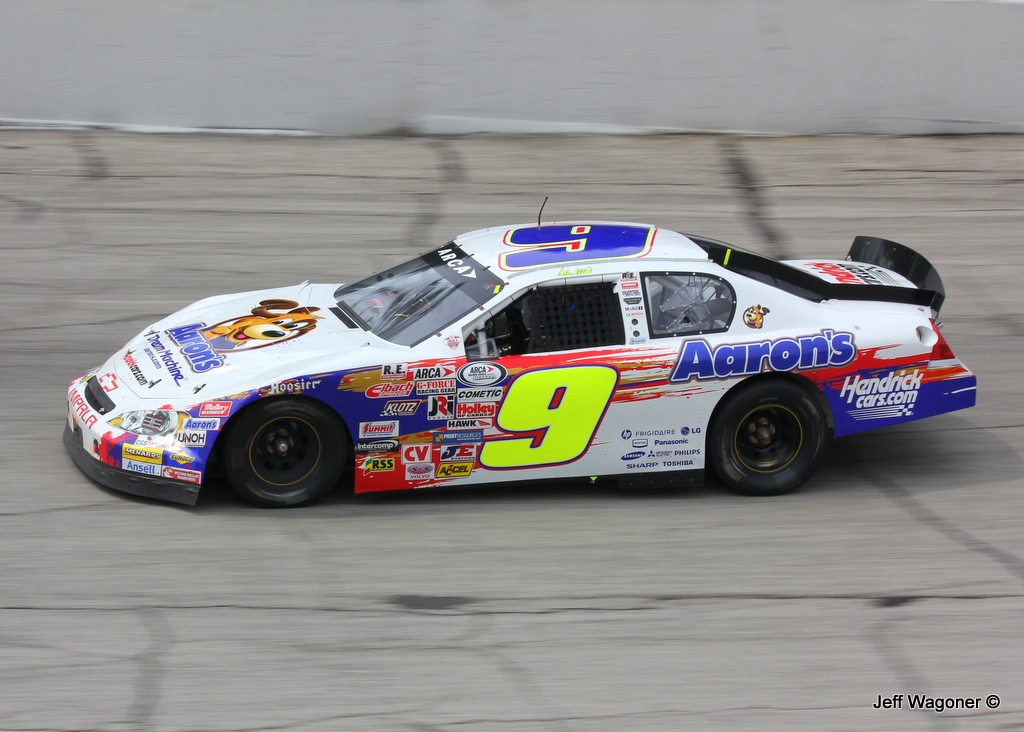This horizontally aligned rectangular image captures a dynamic race car in motion, zooming along a racetrack with a blurry stone wall background. The car, facing left, showcases its left side adorned with vibrant decals and sponsor logos typical of a NASCAR vehicle. Primarily white, the car proudly displays a large yellow number 9 on its side and a blue number 9 on its roof, outlined in red. The car features distinct blue sections near the front wheels and streaks of red near the back wheels. An illustration of a smiling brown dog graces the hood with the word "Aaron's" beneath it in blue lettering. This branding is repeated above the rear wheel and in a smaller version near the front. Additional sponsors, including HendrickCars.com on the lower fender behind the rear wheel, augment the car's livery. The sleek design is completed with black tires that appear to be in motion, accented by yellow outlines on the rims and a black spoiler on the rear left side.